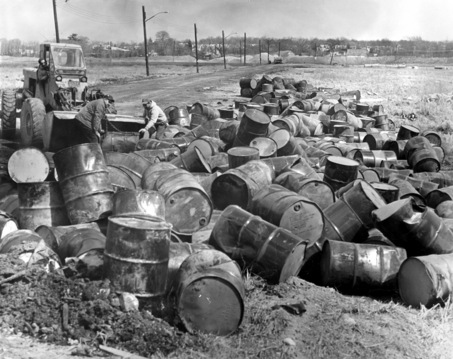In this old, blurry black-and-white photograph, a long gravel road extends into the distance, flanked by telephone poles. Adjacent to the road on the right side, there are mounds of dark-colored metal barrels, many of which are dented and elongated. On the roadside, a large front loader is seen pushing or offloading these barrels, while two men assist by lifting a particularly large barrel. This area appears to be part of a landfill. Fields stretch on both sides of the road, with trees visible in the distant background, and the overall scene hints at a possible industrial or rural setting.